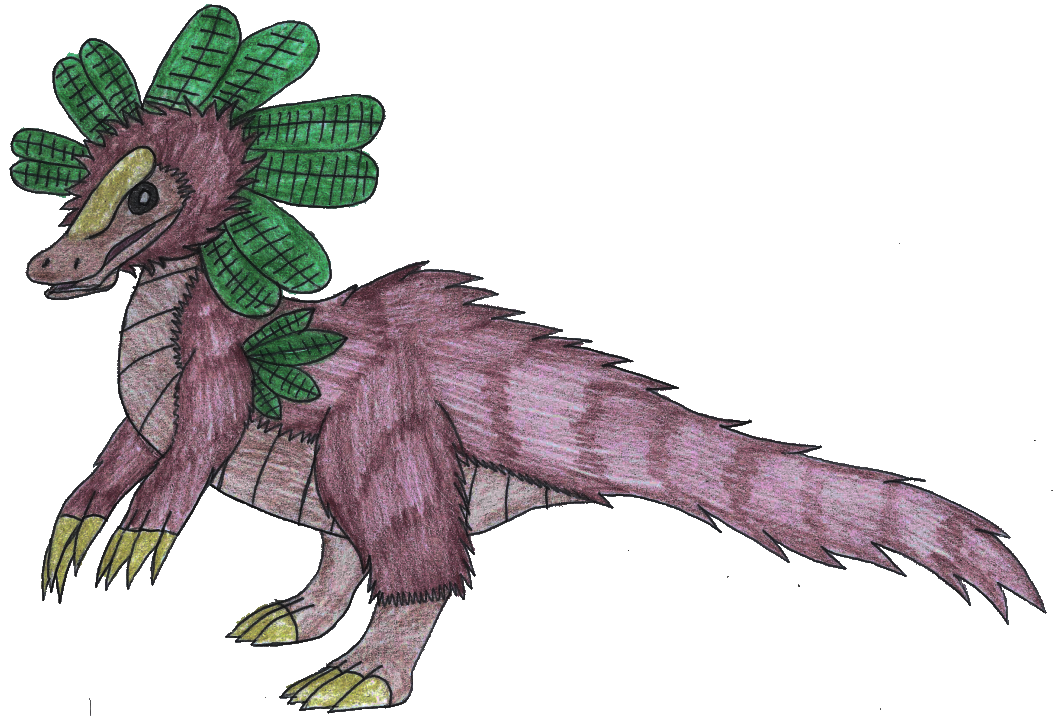The image depicts a creatively drawn, small dinosaur-like creature, likely a fantastical hybrid, made with colored crayons or markers. The creature is covered in a mix of light and darker purple fuzzy fur, particularly around its back, tail, head, arms, and the upper parts of its legs. The lower parts of its legs and its underbelly showcase a smoother texture in a light brown hue, resembling leather. The creature has four prominent, shiny, yellow pointy toes on each foot and similarly colored sharp claws on its hands.

Its head is adorned with a wreath-like arrangement of five sections of double green leaves, each detailed with little lines. Additional green leaves sprout from under its armpits. The face has a strikingly long, alligator-like mouth with a flat, shovel-shaped beak. The top of its head features a unique flat area resembling a shoe print. The creature’s eye is large and black, centered with a whitish-gray dot. Overall, this imaginative drawing blends elements of a dinosaur and a frog, capturing a whimsical and inventive spirit.